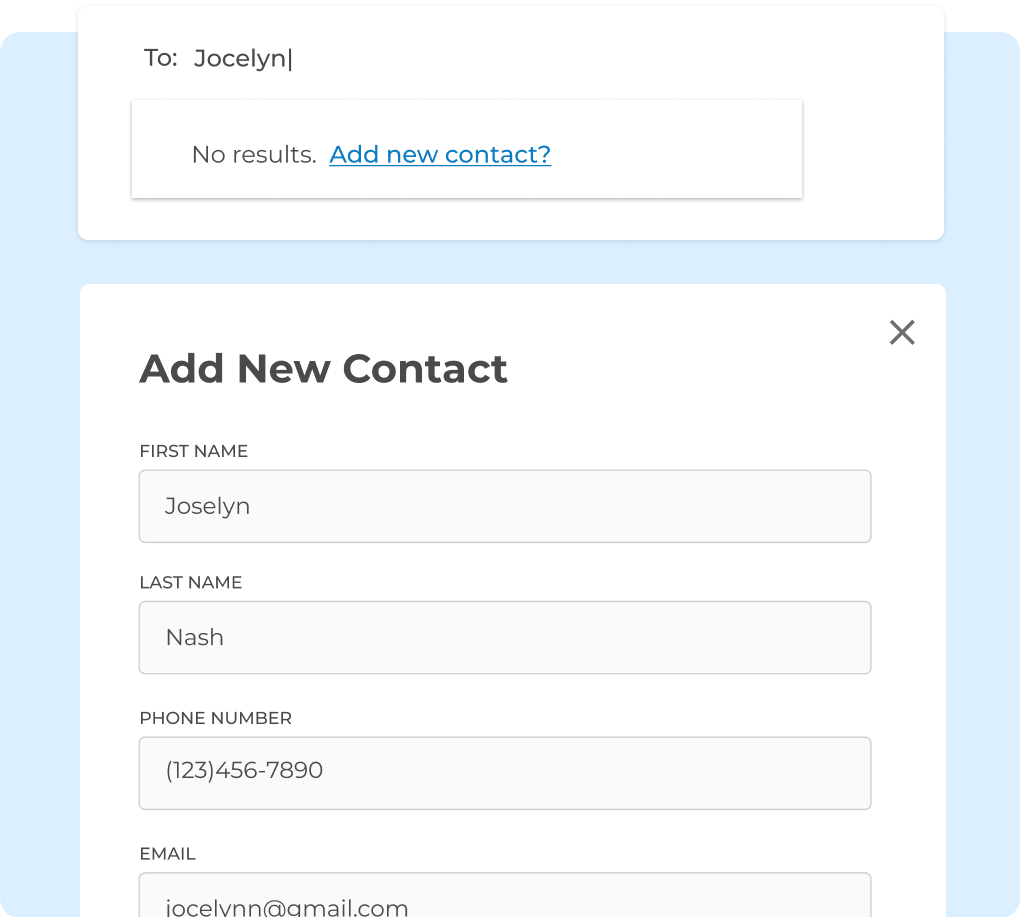The image displays a user interface with a series of rectangular sections in varying colors. At the top, there is a large white rectangle containing the number "2" and the name "Jocelyn." Below this, there is a blue rectangular area which is partially obscured by another white rectangle that reads "No results," framed with a gray outline. Additionally, this section contains a blue link-like text saying "Add a new contact?" indicating an interactive option.

Further down in the interface, within the blue section, another smaller white rectangle is visible, labeled "Add new contact," with an "X" icon on the right side for closing or dismissing this input form. Within this section, fields for entering contact information are displayed. These fields include "First Name," populated with "Jocelyn," "Last Name," filled with "Nash," and "Phone Number," formatted as "(123) 456-7890." The "Email" field shows an address partially cut off at the bottom, reading "jocelyn@gmail.com."

The design suggests that the blue rectangle, which is partially hidden by the overlying white sections, resembles the shape of an "H." The layout and formatting indicate a contact management interface, likely part of a software or application designed to add and manage contact information.